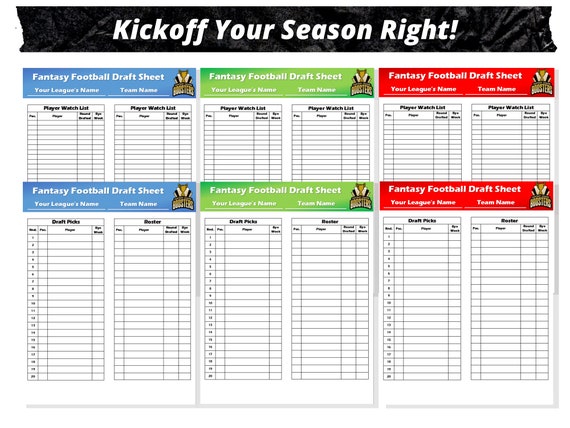The image showcases digitally drawn fantasy football draft sheets organized within a wide vertical rectangular frame. Dominating the top portion is a horizontal black stripe featuring the motivational slogan "Kick off your season right" in italicized white font. Beneath this stripe, the main background is white and divided into three distinct columns, each containing two vertically arranged draft sheets with contrasting color-coded headers.

The first column, situated on the left, displays two draft sheets with blue headers, while the middle column houses sheets with green headers, and the rightmost column features red headers. Each draft sheet consistently bears the title "Fantasy Football Draft Sheet," followed by placeholders for "Your league's name" and "Your team name." Below these titles, the sheets are sectioned into organized, spreadsheet-like segments. The upper segments are reserved for "Player Watch List," catering to tracking potential draftees, whereas the lower sections, though less readable, appear to be allocated for draft picks and roster management.

All these sheets, regardless of their header color, incorporate black fonts for the chart details, set against a primarily white paper-like background. The neat division of columns and categorization provides a comprehensive tool for fantasy football enthusiasts to meticulously plan and manage their team selections.